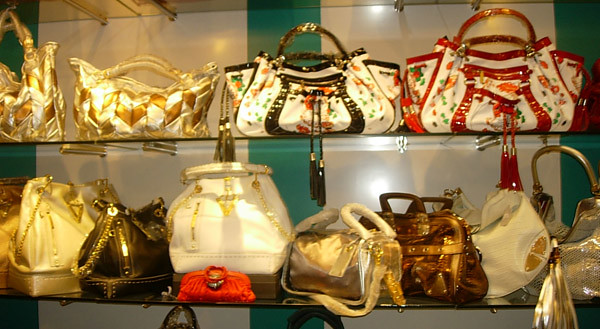This photograph captures a vibrant and ornate display of vintage or antique women's handbags, though men could use them too, arranged on glass shelving with subtle overhead lighting, giving it a museum-like or exhibit feel. The display is set against a mostly white wall featuring multiple vertical green stripes, drawing attention to the colorful array of bags. On the top shelf, there are four large handbags: two shiny metallic ones with gold and white chevrons, a floral-patterned bag with red trimming, and another similar floral bag with black edging. Below, the shelf is cluttered with nine additional handbags, comprising white, ivory, black, brown, and silver variations. Noteworthy among them is a small red clutch bag. The handbags are notably flashy, gaudy, and intricate, with bold and colorful designs that indicate their ornate and possibly expensive nature.